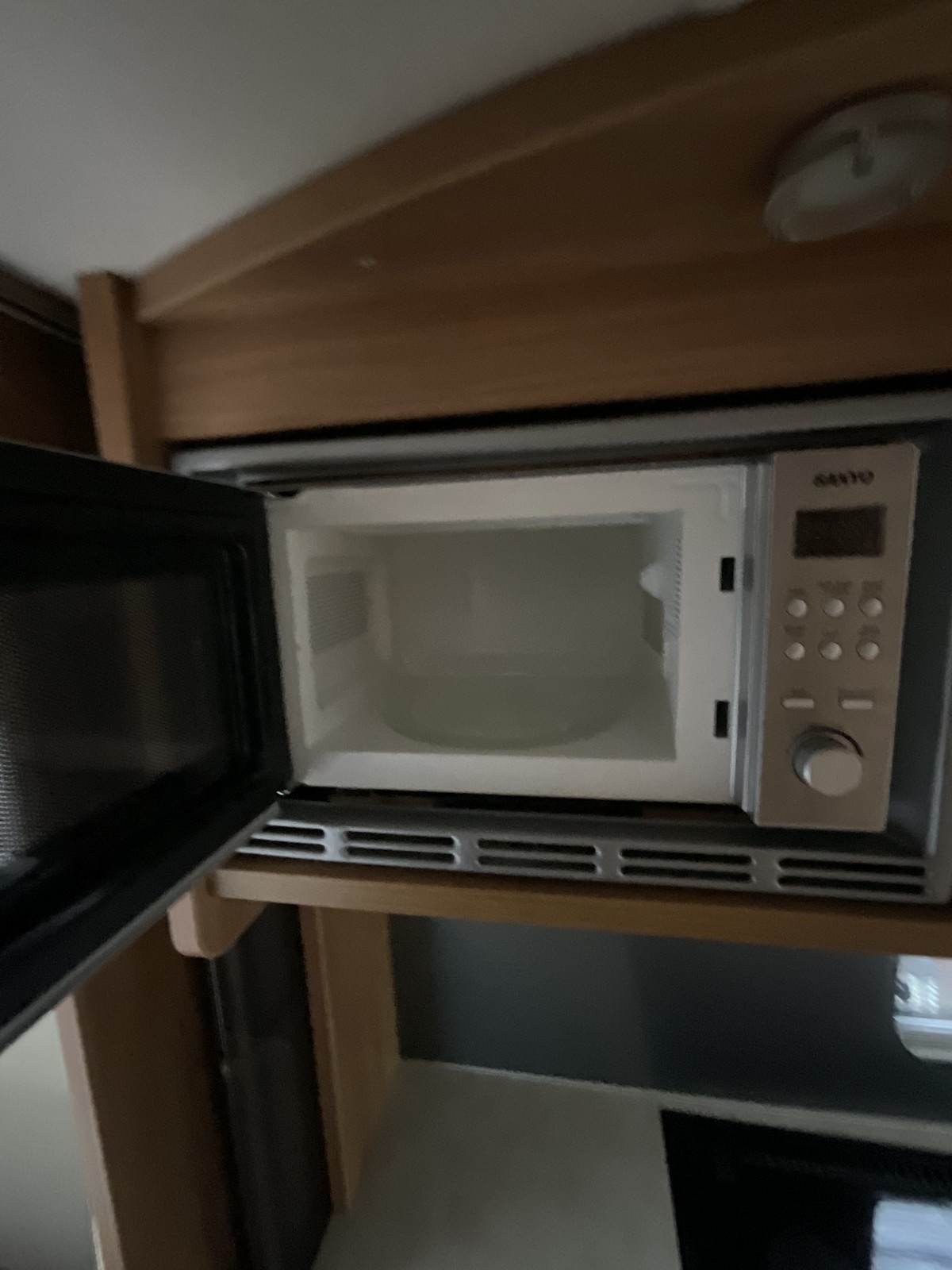The photograph depicts a compact Sanyo microwave built into a wood-grain wall inside what appears to be a camper or RV. The microwave's door, which is black on the inside, is open to reveal a white interior and features a silver control panel. Above the microwave is an arched wooden panel. A small countertop and a glimpse of a rounded corner window are visible beneath the microwave, further suggesting the setting of a camper or RV. The overall lighting is dim, contributing to a slightly dark and out-of-focus image. Various colors can be seen in the photo, including tan, brown, white, black, and gray, with the microwave centrally located and an overhead light in the top right corner.